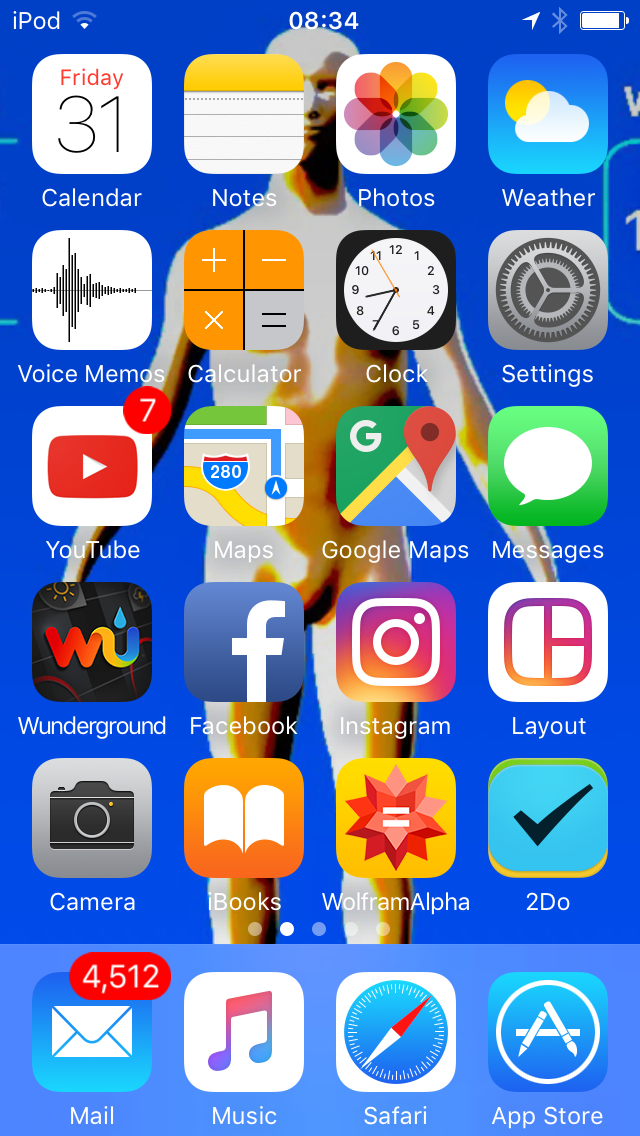The image captures the front display of an iPod with a detailed arrangement of apps and notifications. In the upper left corner, the word "iPod" is prominently displayed in white letters. The top center shows the time "08:34" along with an arrow indicator and the battery icon.

The main screen features a variety of app icons arranged in a grid pattern. The first row includes Calendar, Notes, Photos, Weather, Voice Memos, Calculator, Clock, and Settings apps. The second row displays YouTube with seven unread notifications, Maps, Google Maps, Messages, WonderGram, Facebook, Instagram, Layout, and Camera apps. The third row contains Books, an app labeled "William Alpha," and To Do.

The background of the display is a striking blue with an interesting abstract image of a person's body, which is partly flesh-colored and partly illuminated in white, resembling light beams. At the bottom of the screen, a lighter blue section shows additional app icons for Mail, Music, Safari, and the App Store. The Mail app has a red notification badge indicating 4512 unread emails. 

Overall, the image presents a well-organized and vibrant home screen on the iPod, set against a visually captivating background.